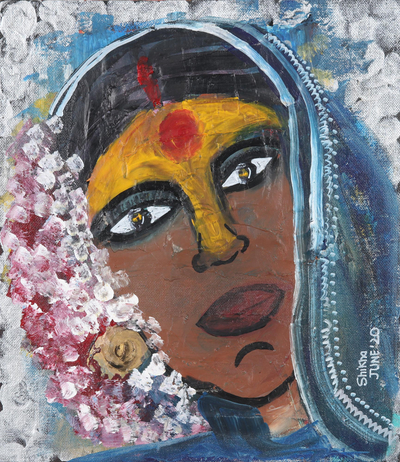This artwork, executed in watercolors, vividly portrays a woman's face turned at an angle, with her head inclined from the upper left to the lower right of the canvas. The woman's face features a striking yellow hue on her forehead that extends down towards the brow and the bridge of her nose. A distinct red dot is prominently placed between her eyes on her forehead, adding a captivating focal point to the composition. She is adorned with a blue headpiece that gracefully contrasts with the warm tones of her skin, further accentuating the delicate yet expressive nature of the painting.